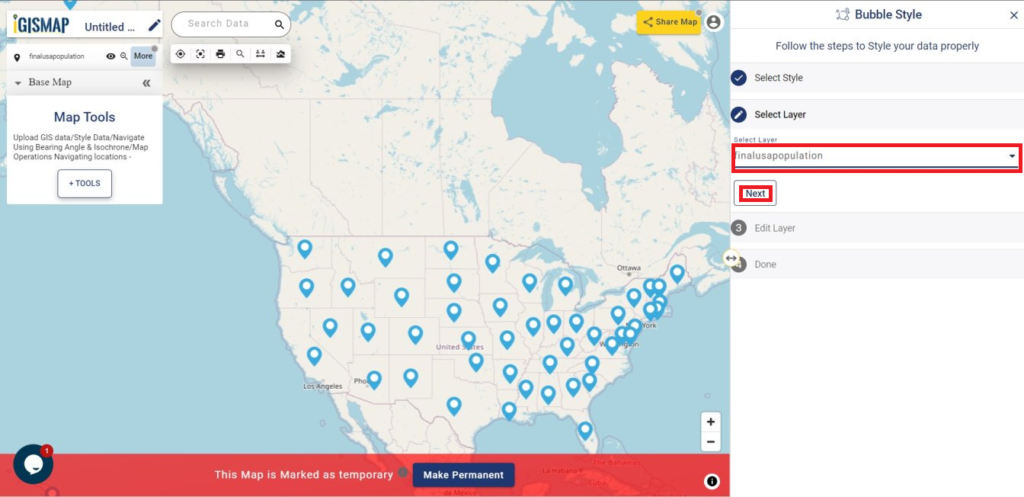The image is a detailed view of a GIS map interface. 

In the top left corner, there is a white rectangular section extending horizontally. This section contains the title "GIS MAP" on the left side and the word "Untitled" to the right of it. A pencil icon, presumably for editing, is situated at the far right of this rectangular section.

Beneath this header, there's text reading "Final US Population" followed by "Base Map," which includes a dropdown menu indicated by a downward arrow. To the right, there are arrows for navigation.

Below this, a section labeled "Map Tools" lists several functionalities: Upload GIS Data, Style Data, Navigate Using Bearings, Angles, and Isochrone, and Map Operations, which includes Navigating Locations. A button labeled "Plus Tools" is also present here.

To the right of the "GIS MAP" title is a search field containing the placeholder text "Search Data" in gray along with a search icon.

The main portion of the image shows a map of the United States dotted with numerous pins indicating various data points. 

On the right side, there’s a small section labeled "Bubble Style" followed by an "X" button. Instructions for styling the data appear as "Follow the steps to style your data properly." These instructions include "Select Style," "Select Layer," and specifically highlight a layer named "LINALUSAPOPULATION," which has both a blue and a red box around it. Another dropdown is available for layer selection.

Finally, there is a "Next" button outlined in red. The overall setup appears to be intended for educational purposes, guiding users through the process of GIS mapping and data styling.